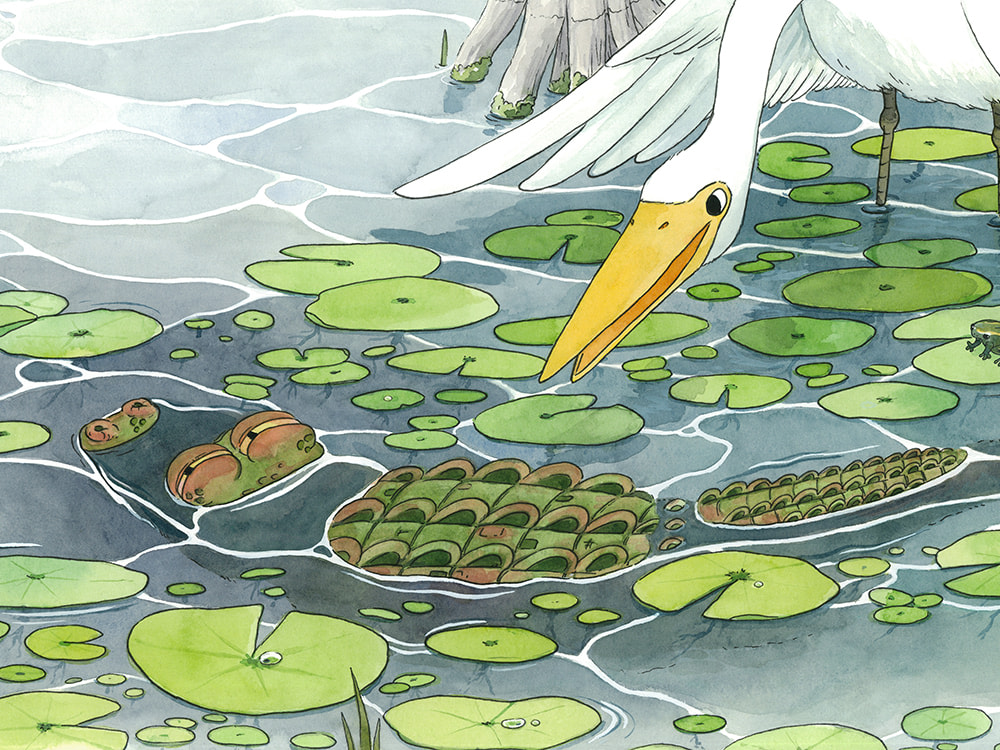In this lively, cartoon-style painting, a large white bird, reminiscent of either a crane or a heron with a strikingly long yellow beak, is depicted in motion. The bird, which has a serene expression, is poised over the water with its wings slightly visible behind it. The scene is set in what appears to be a vibrant swamp or pond, teeming with life and movement. Lily pads float on the water's surface, some hosting small frogs, adding to the whimsical nature of the artwork. Amidst the floating reeds and roots, likely from a sprawling cypress tree in the background, a crocodile begins to emerge, its eyes and ridged back breaking the water’s surface. The entire scene is further enriched by a spread of dishes that include what appear to be wraps and other meals on a makeshift banquet table, suggesting a playful atmosphere where the bird seems to be inspecting or perhaps contemplating a bite. The artwork is imbued with a sense of daylit tranquility, blending natural elements with a touch of imaginative charm.